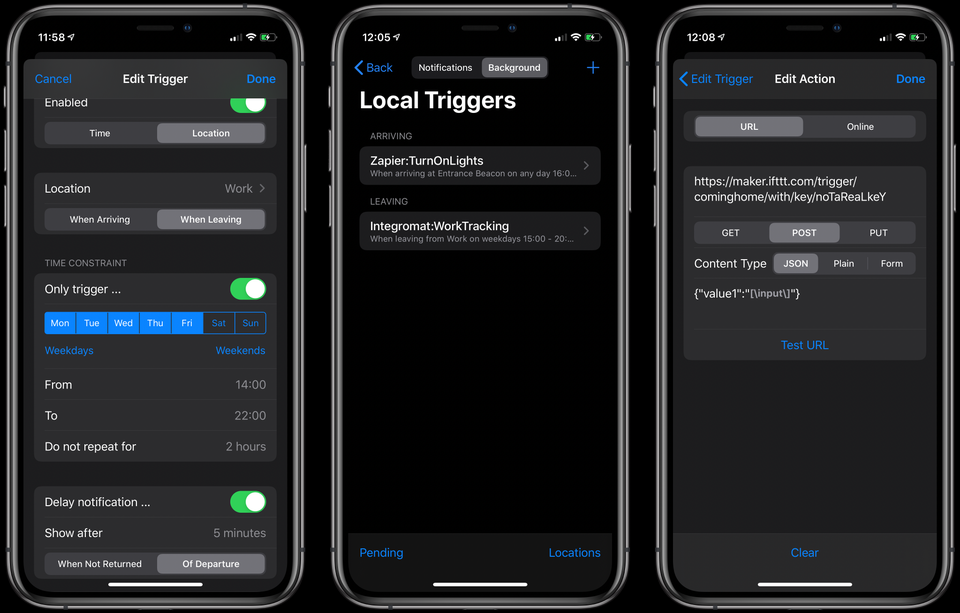The image comprises three separate smartphone screens, each displaying different settings and actions for a trigger-based automation app.

**First Screen:**
- **Header:** "Edit Trigger" with a blue "Cancel" button on the left and a blue "Done" button on the right.
- **Status Section:** "Enabled" indicated by a green icon.
- **Conditions:**
  - **Time & Location:**
    - **Time Constraint:** "Only trigger" is turned on.
    - Days: Monday through Friday ("weekdays").
    - Time: From "14:00" to "22:00".
    - Additional Note: "Do not repeat for two hours."
    - Option: "Delay notification" is turned on, showing notifications after five minutes.
    - **Location:** "Work".
      - Two options: "When arriving" and "When leaving."
- **Summary:** Set for departure under specific time and location constraints.

**Second Screen:**
- **Header:** Blue "Back" button.
- **Notifications & Background Section:**
  - **Arriving Action:** "Zapier" integration is set to "Turn on lights when arriving at the entrance beacon" on any day.
  - **Leaving Action:** "Integrates Work Tracking" when leaving work on weekdays at 15:00.

**Third Screen:**
- **Header:** "Edit Action" with a blue "Edit Trigger" button and a blue "Done" button.
- **Action Details:**
  - **URL or Online Option:** A URL has been entered.
    - **Request Type:** "POST."
    - **Content Type:** JSON.
  - Buttons:
    - Blue "Test URL" button.
    - Blue "Clear" button at the very bottom.

This comprehensive overview demonstrates a robust automation setup involving time-specific and location-based triggers, accompanied by actions that interact with external services and APIs.